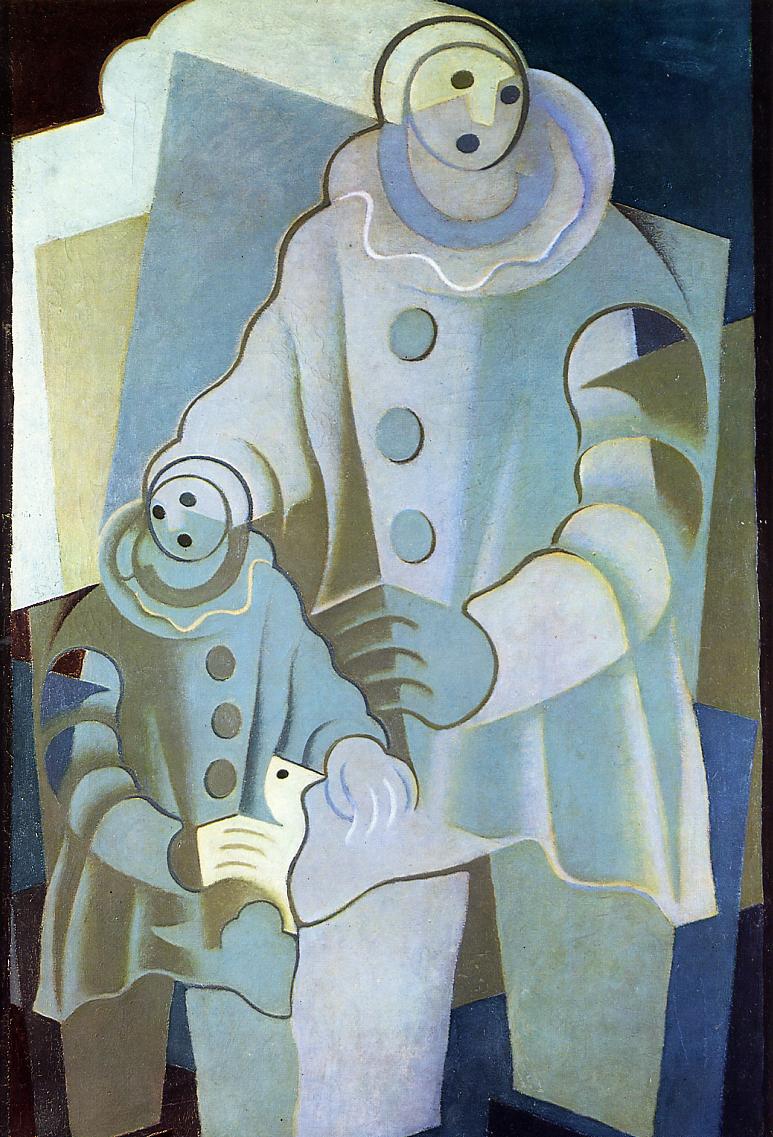The painting is a highly abstract and esoteric piece of art, depicting two ghost-like figures dressed in long tunics reminiscent of clown suits, characterized by their white cloth-covered heads with three black dots forming minimalist facial features. The larger figure, towering over a smaller, child-like counterpart, both wear garments adorned with three buttons and have collars that hint at clown attire. The taller figure supports the smaller one with its hands resting on the child's arm and back, conveying a sense of closeness and protection. The child is holding a small, white four-legged animal, possibly a toy horse. The background features a blend of various shapes and patterns, including rectangles and trapezoids that seamlessly merge with the figures’ forms, and a mix of colors—light purple, turquoise, and shades of blue—accentuated by square patterns in gold and white, giving the scene a strikingly modern yet oddly dimensional feel.